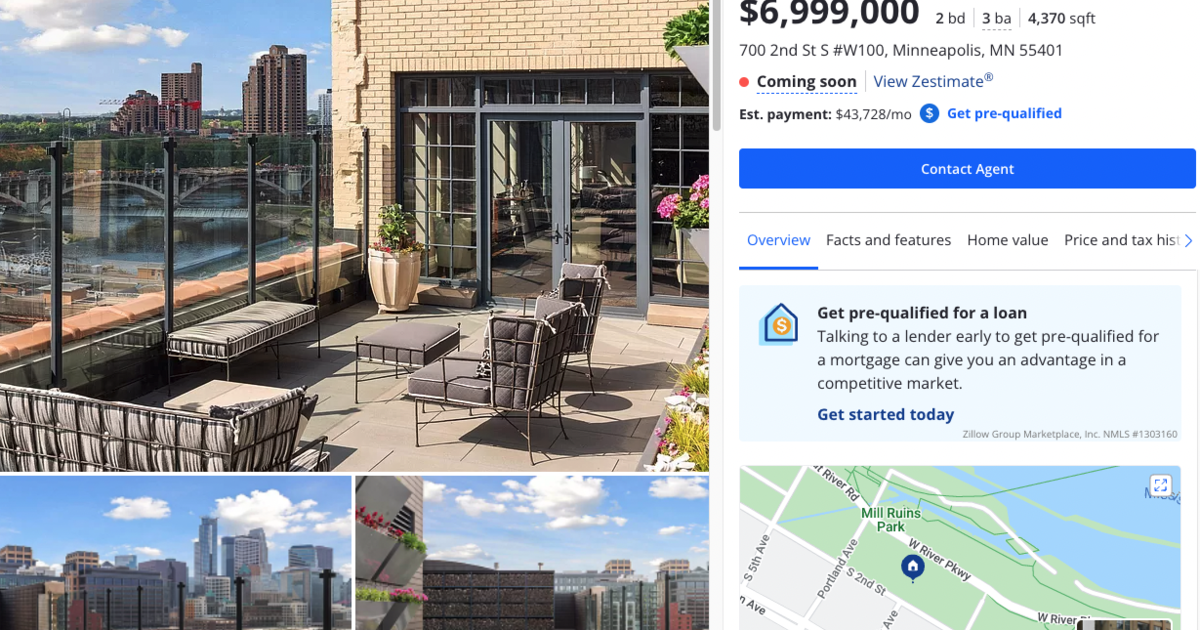For Sale: Luxurious Home at $6,000,999 located at 702 2nd Street, Southwest Unit 100, Minneapolis, Minnesota, 55401. The property boasts two spacious bedrooms, three modern bathrooms, and an expansive living space of over 4,700 square feet. The listing features a detailed map for easy navigation, three high-quality images showcasing the property’s elegant interiors and well-maintained exterior. Prospective buyers are encouraged to contact the agent for further inquiries and to get pre-qualified for a loan. The charming home is complemented by well-manicured lawns and is situated in a picturesque neighborhood with convenient access to nearby roads and amenities. This advertisement highlights the premium aspects of the home, inviting serious interest from potential buyers.